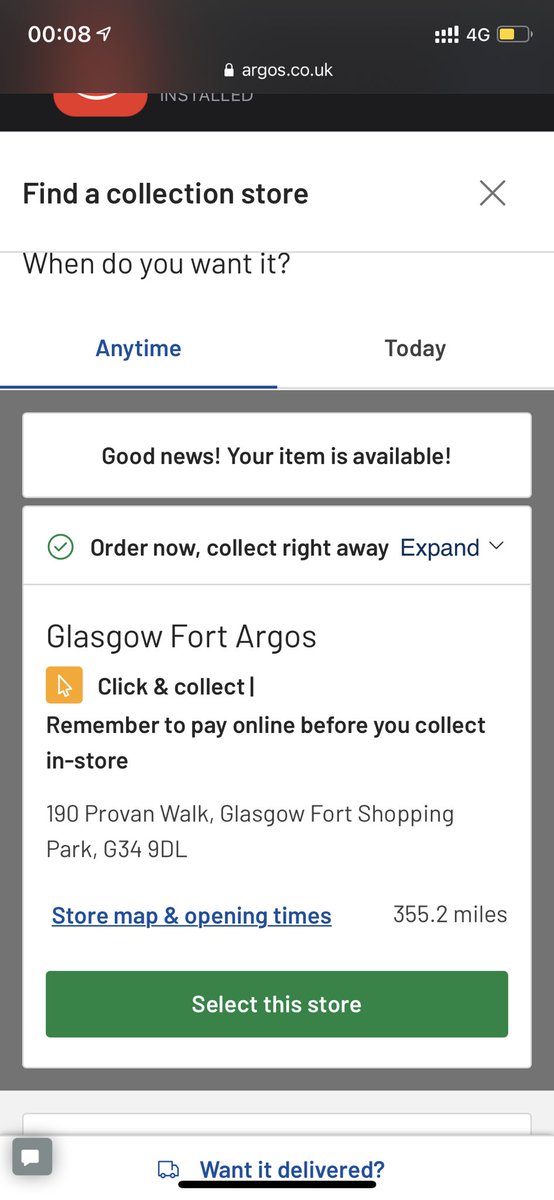Screenshot of an iPhone displaying a webpage from augles.co.uk at 12:08 AM, with a half-full battery and 4G network. The interface shows a white background with multiple elements:

Top Section:
- To the left, there's "Find a collection store" with an adjacent "X" button.
- Above is a partially visible "Install" option featuring what appears to be the Pinterest icon.

Main Content:
- Below a thin black line, there is the prompt "When do you want it?" followed by "Anytime" and "Today" on the same line.

Middle Section:
- A gray-bordered box with:
    - "Good news, your item is available."
    - A green checkmark.
    - "Order now, collect right away" with an expandable dropdown arrow.
    - Details: "Glasgow, 4th August" with reminders to "click and collect" and to "pay online before you collect in store."
    - Address: "190 Proven Walk, Glasgow 4th Shopping Park, G3490L."
    - Link for "store map and opening times" in blue text.
    - The distance is "355.2 miles."
    - A green bar option to "Select a store."

Bottom Section:
- Below the gray border, in blue text with a delivery truck icon, there is "Want it delivered?" and a message button likely for email or online chat.

This detailed flow guides users through collecting their item, providing all necessary options, locations, and additional instructions.